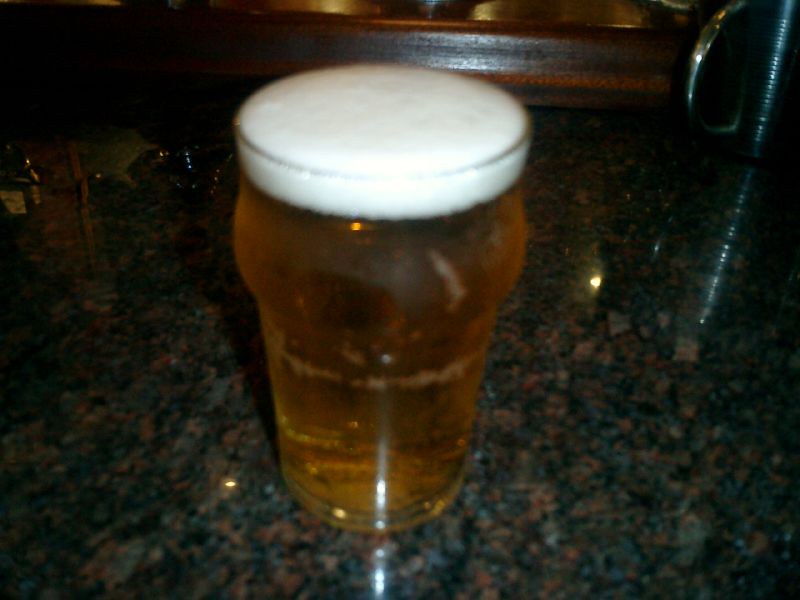The photograph captures a pint glass of medium amber beer, filled to the top with about an inch of white foam. The glass has a slight outward curvature near the top before tapering inward again and is positioned directly in the center of the image. The beer is on a dark speckled stone counter that includes flecks of green, gray, black, and tan. Bubbles are visible within the beer, and a metal cylindrical object is placed nearby on the counter. In the background, you can see a medium brown wooden ledge, suggesting the setting might be indoors, possibly in a bar at night. Lights are reflecting off the counter surface, enhancing the detail and texture of the scene.